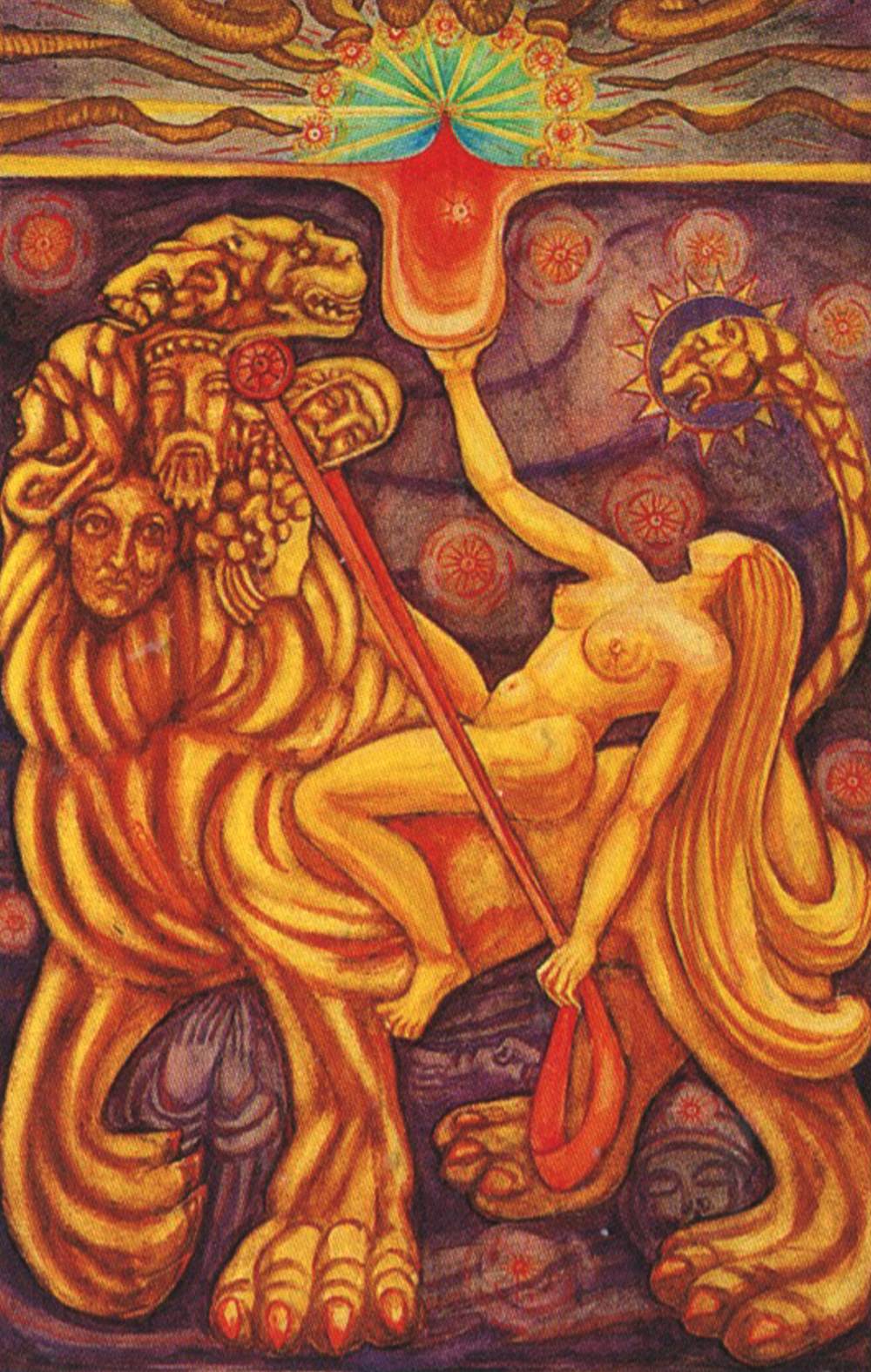This vibrant painting, awash in shades of gold, orange, red, and accented with purples, blues, and greens, features a striking tableau. At its center is a naked woman with long, flowing hair, prominently displaying her breasts. She is straddling a fantastical creature that appears to be a fusion of a lion, panther, and griffin, with its body adorned with swirling muscles and wavy fur. Uniquely, the creature has multiple human-like faces, including those of men, and possibly a wild animal, embedded within its head.

The woman gazes upwards toward the sky; in her left hand, she holds red reins or a scabbard that extend toward the beast's head. In her right hand, she raises an object that is glowing and surrounded by a multicolored, star-like orb in teals, golds, and reds, with ribbons emanating from it. Above her, a gold and brown striped serpent stretches skyward, culminating in a sun-like structure around its head.

Beneath the creature she rides, shadowy figures in dark purples are either prone or sitting, adding an eerie depth to the scene. The painting masterfully blends elements of fantasy and surrealism, creating a richly detailed and dynamic visual narrative.